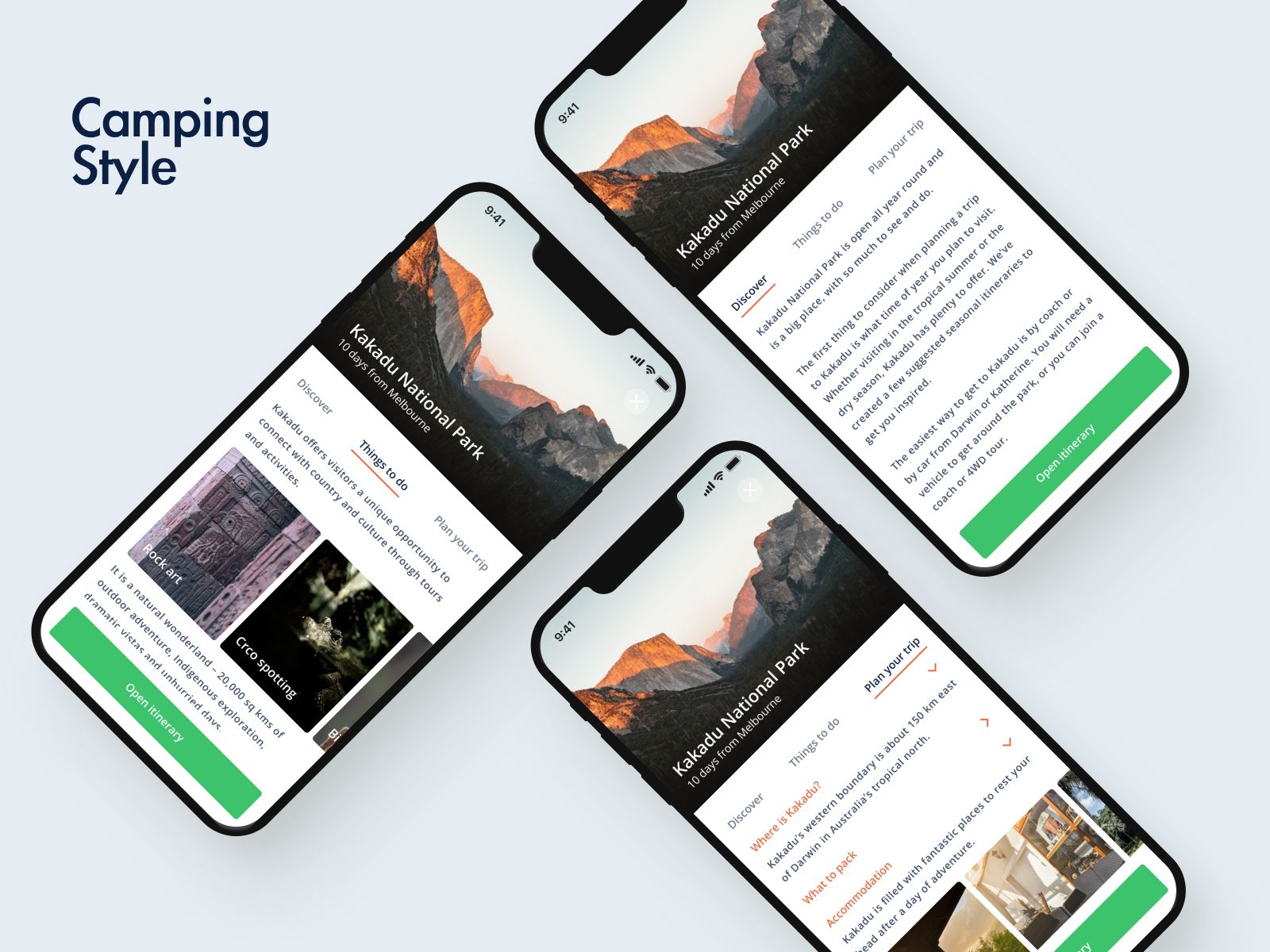This advertisement showcases a phone application or website tailored for exploring Kakadu National Park, displayed against a very light blue background. The upper left corner prominently features the phrase "Camping Style" in blue font. The ad highlights three smartphones, each demonstrating different features of the app.

1. **Top Right Phone**:
   - **Tab**: Discover.
   - **Content**: Contains detailed text about the mountain, although the text is too small to be clearly read.
   - **Button**: A green "Open Itinerary" button at the bottom.

2. **Top Left Phone**:
   - **Tab**: Things to Do.
   - **Content**: Displays various images of activities available at Kakadu National Park, with visible labels such as "Rock Art" and another partially readable activity, possibly "Wildlife Spotting."
   - **Button**: A green "Open Itinerary" button at the bottom.

3. **Bottom Right Phone**:
   - **Tab**: Plan Your Trip.
   - **Content**: Features several orange drop-down menus that allow users to plan different aspects of their trip.

This comprehensive view of the app's different functionalities emphasizes ease of discovering information, exploring activities, and planning a trip to Kakadu National Park.